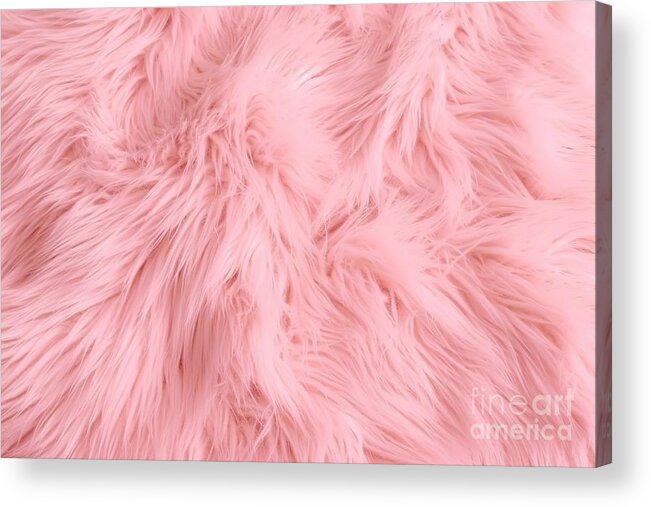The image captures a close-up photograph of a light pastel pink fur rug with intricate waves of curves and curls, giving it a shiny and fluffy texture. The photo, possibly depicting a piece of artwork made to look like a 3D-printed image, is slightly tilted to the side and set against a white background with notable shadows, enhancing its three-dimensional appearance. The bottom right corner of the artwork's frame is visible, bordered by thick white strips both horizontally at the bottom and vertically on the right. In this corner, the white text "Fine Art America" can be seen. The soft, seamless look of the long pile animal fur, ideal for a baby's room, dominates the image with its fake fur texture.